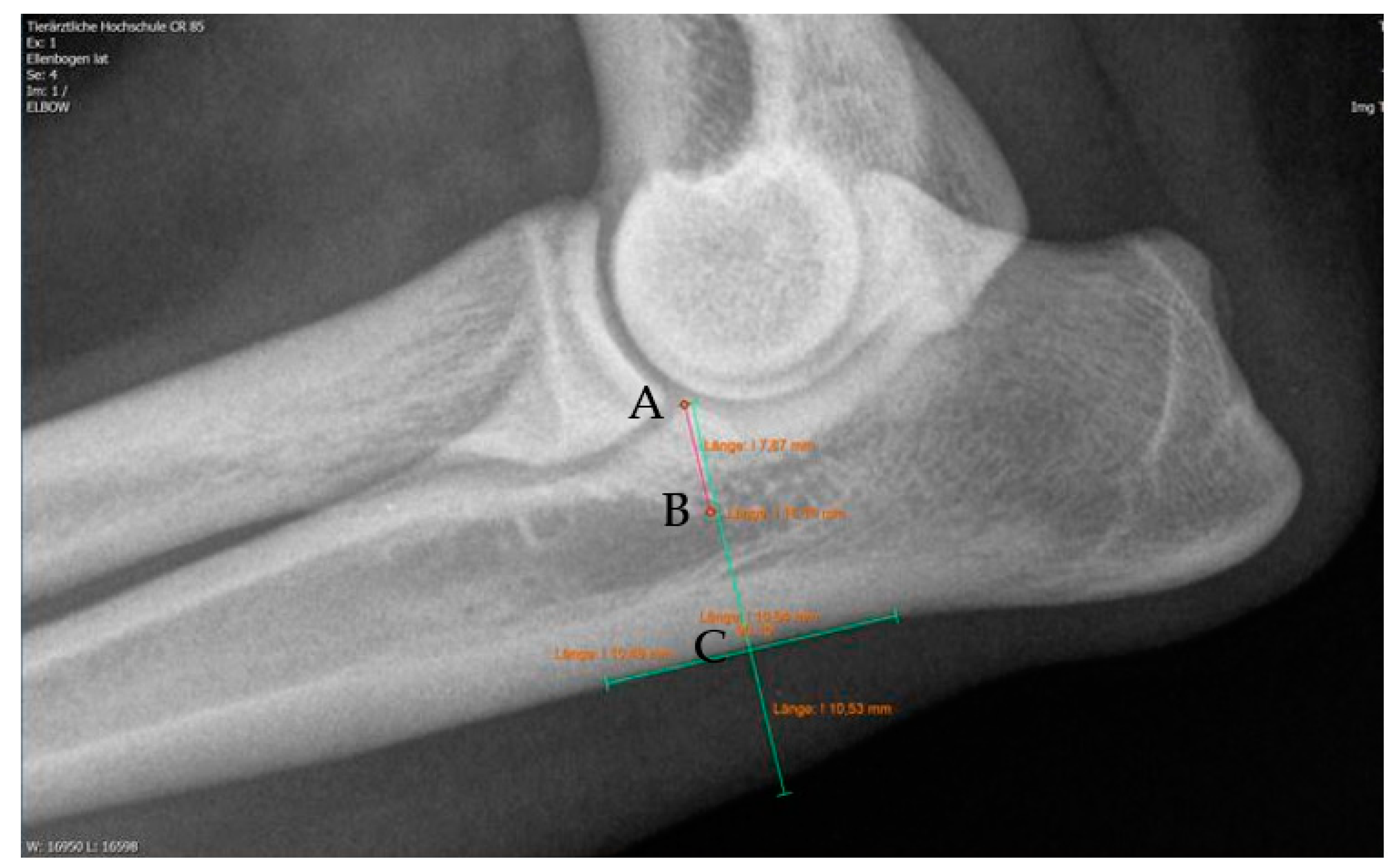This is a close-up x-ray image, likely a photograph or scan, showcasing an elbow joint. The central focus is on the area where the bones and joints connect. Marked prominently in black lettering are labels A, B, and C, situated from top to bottom along the elbow joint. Additionally, there are orange and turquoise lines, possibly indicating measurements, with dots and lines connecting these points to respective labels. In yellow lettering, specific sections of the bone are annotated with millimeter measurements, detailing the lengths of certain bone parts. The image also features some partially legible text: in the top left corner, a label referencing the elbow, and in the bottom left corner, a series marked W and L followed by numbers. In the top right corner, there is cut-off text that reads "image." Overall, the x-ray has a slightly compressed and unclear quality, adding to the challenge of reading all the annotations and measurements.